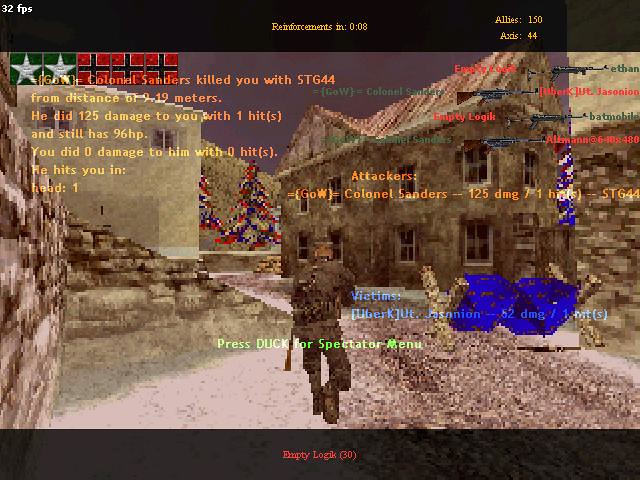This is a detailed screenshot from a battle royale action-shooter game. In the upper right-hand corner, there are four images of guns, each oriented towards the right. These gun icons are outlined with red text, although the specifics are difficult to make out. Dominating the lower center of the image is a figure of a soldier, standing poised and ready for action. Additionally, in the upper left-hand corner, there are several red blocks, possibly indicating health, armor, or another game-related metric. The overall composition suggests an intense, tactical scenario within the game.